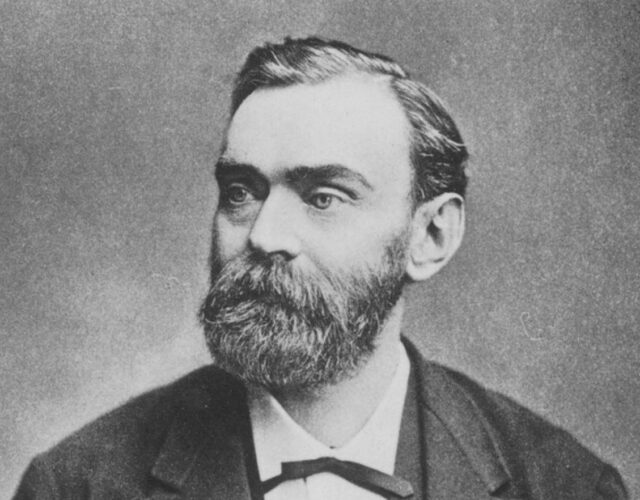This black-and-white portrait presents a famous 19th-century man with dark hair parted to his left. He has a thick, well-trimmed full beard and mustache so long it obscures his mouth. He gazes off to his right, allowing a view of his full face, not just his profile. The photograph is taken from the shoulders up, showing a distinguished appearance with a neatly tied ribbon-style bow tie around his neck, a white collared dress shirt, and a layered ensemble featuring a black vest under a dark, notch-collared suit jacket. The background is plain gray, adding to the old-fashioned, solemn atmosphere of the image. His eyes appear gray, adding a striking contrast to his dark hair and attire.